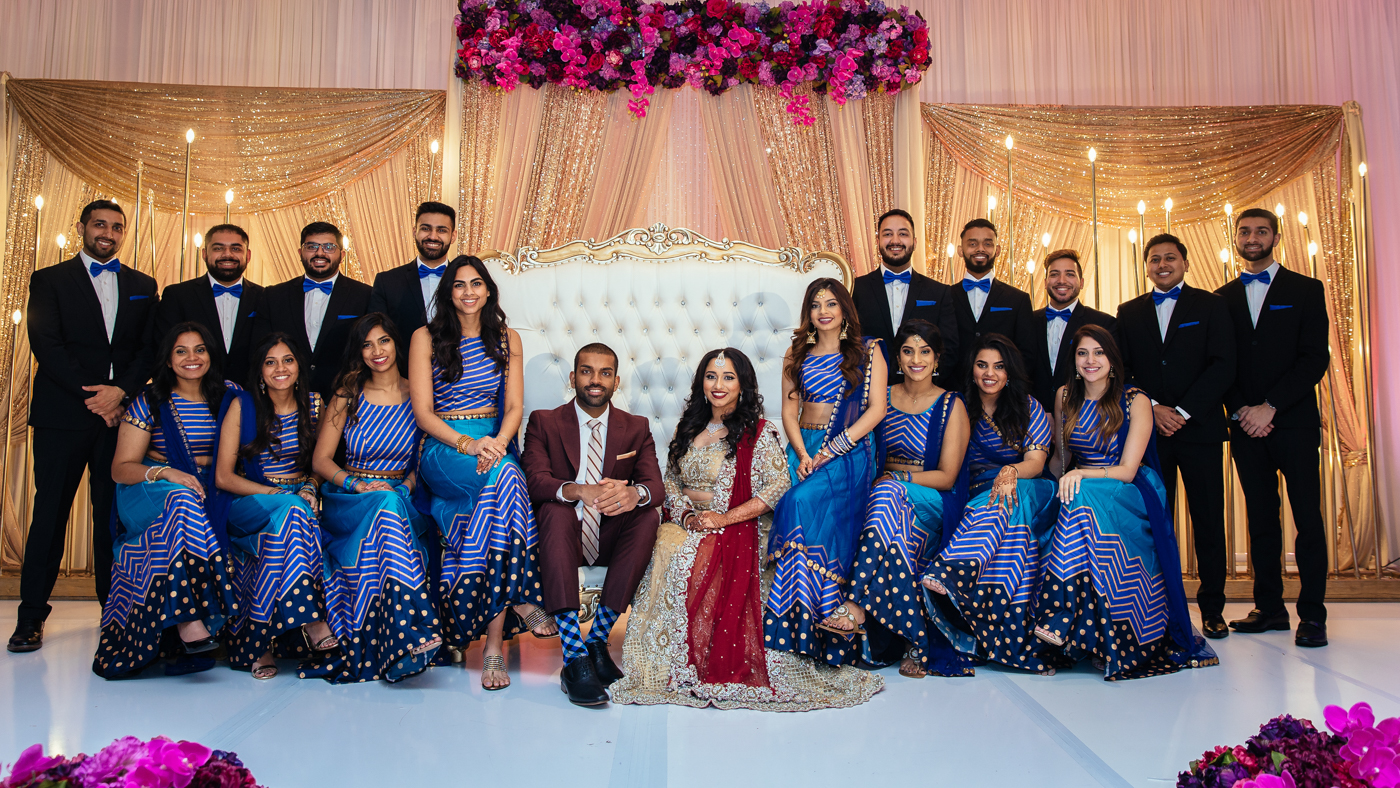This horizontal rectangular image captures an ornate, East Indian themed wedding celebration with a large wedding party. At the center of the photograph, a bride and groom are seated on an elaborate white and gold Louis XIII style couch upholstered in white fabric. The bride, wearing a long taupe dress adorned with white jewels and intricate floral designs, has a jeweled pendant on her forehead, a thick diamond necklace, a red scarf draped around her shoulders, and henna tattoos decorating her hands. Her long, dark, curly hair complements her traditional and ornate attire. Beside her, the groom is dressed in a dark burgundy suit with a white button-down shirt and a white and burgundy striped tie, pairing his attire with blue, white, and black checkered socks and black shoes.

Flanking the couple are the wedding party members, with four bridesmaids and four groomsmen on the bride's side, and four bridesmaids and five groomsmen on the groom's side. The bridesmaids, all sporting long dark hair, wear matching blue and gold striped dresses with dark blue trim and gold circular patterns, and shawls around their shoulders. Standing behind each bridesmaid, the groomsmen are dressed in black tuxedos with blue bow ties.

The backdrop features opulent wedding decorations with sparkling gold drapes and hanging curtains adorned with rows of purple and red flowers. This beautifully crafted setting, coupled with the intricately dressed participants, highlights the cultural richness and joyous atmosphere of the celebration.